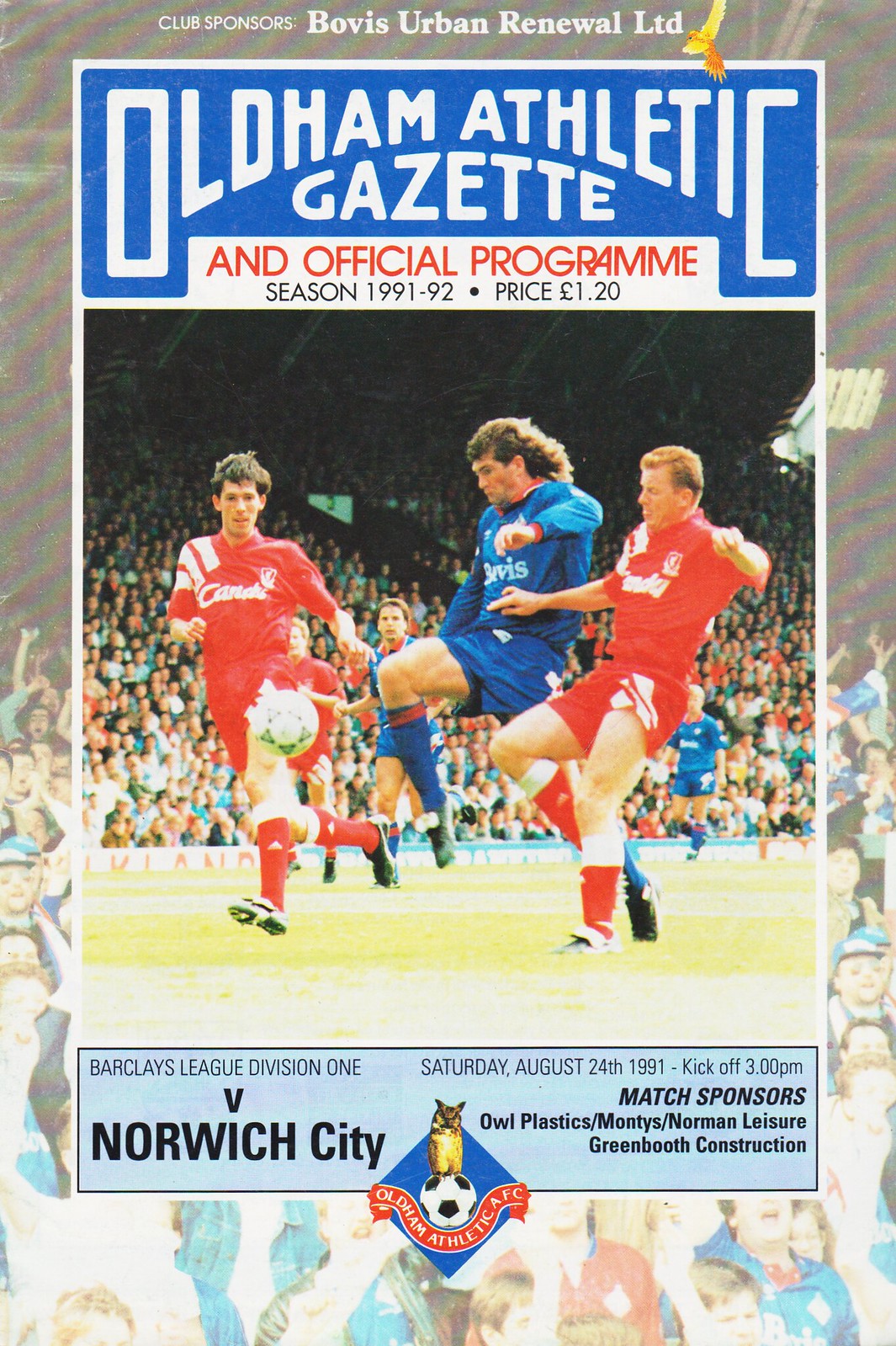This image is the front cover of an official match program titled "Oldham Athletic Gazette" for a soccer game in the Barclays League Division 1, held on Saturday, August 24, 1991, with kickoff at 3 p.m. Designed with a gray background accented by wavy red lines, the cover prominently displays a full-color photograph of a match in action. In the photo, two players in red flank a player in blue who is in the act of kicking a soccer ball, with additional players and a large audience visible in the background. 

At the top of the cover, "Club Sponsors: Bovis Urban Renewal Ltd." is written in small white font. Just below, there's a square section where "Oldham Athletic Gazette" appears over a blue background, with "an official program" beneath it in red over white. The season indicated is 1991-1992 and the price listed is £1.20. At the bottom section, it notes the match against Norwich City, with sponsors Owl Plastics and Green's Booth Construction, as well as Monty's Norman Leisure. An "Oldham Athletic FC" logo featuring an owl on top of a soccer ball completes the design.